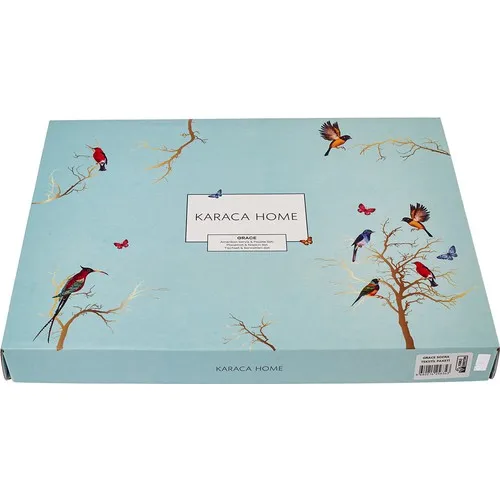This image features a very decorative, rectangular box set against a white background. The box is a beautiful medium shade of blue and prominently displays "KARACA HOME" in a white square in the center, with an additional unreadable square underneath and the same branding on the side. The front of the box is adorned with an artistic depiction of bare trees populated with various birds and butterflies. Birds include a red bird perched on the left branch, a blue jay, a robin, and a more exotic bird with a long beak and tail on the lower left. A golden and black bird is depicted in mid-flight towards a branch on the top right. Surrounding the trees are butterflies, including a red butterfly and a blue butterfly in the center. On the right-hand side of the box, there is a barcode.